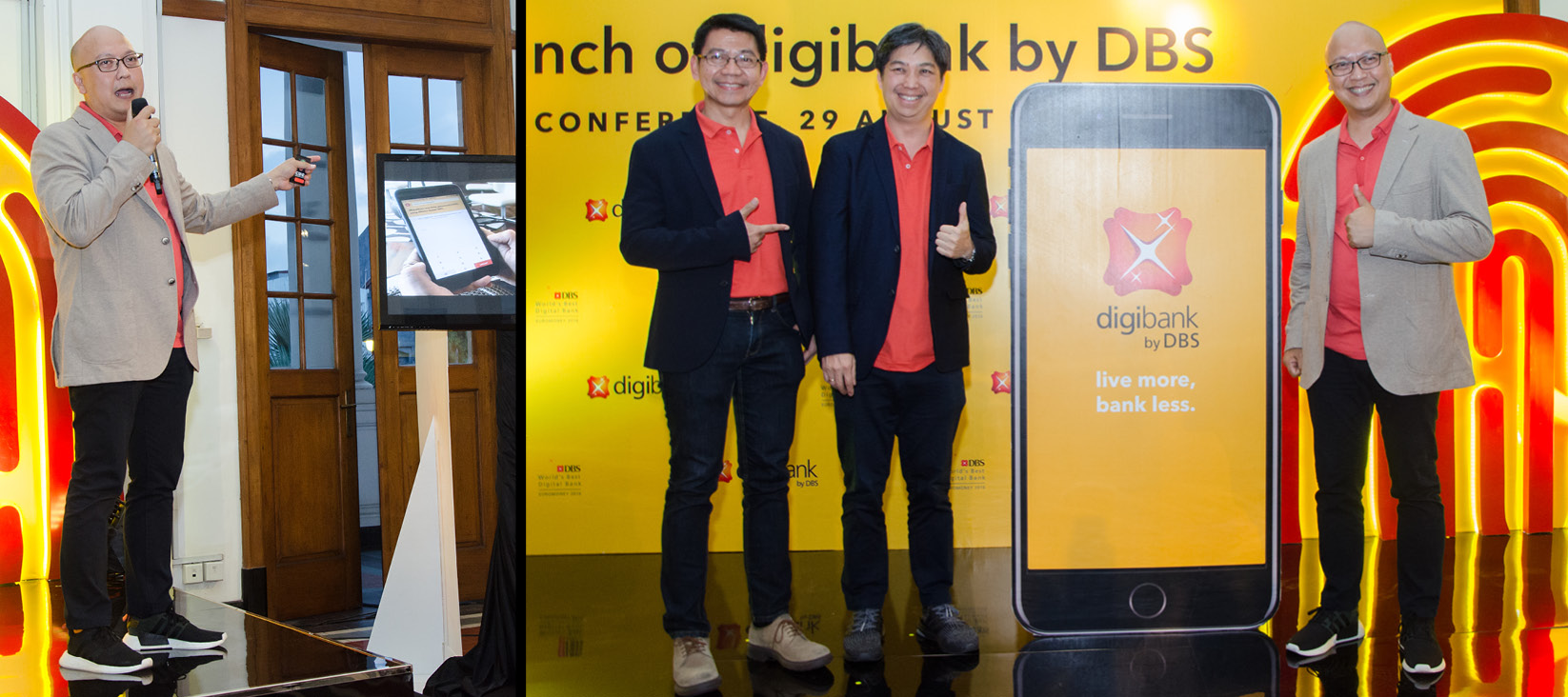The photo captures an engaging event dedicated to promoting the Digibank by DBS mobile app. Dominating the center of the image is an oversized smartphone cutout displaying the Digibank by DBS logo and the tagline "Live more, Bank less." Positioned to the left of this cutout are two men dressed in black blazers with bright red shirts underneath, each sporting black pants. One of them, who is wearing black framed glasses, is holding a microphone in his right hand and gesturing towards a screen showing a tablet presentation. Further to the left, beyond a brown glass-panel door and a curtain, the same gentleman appears again, actively pointing at the screen. To the right of the oversized phone cutout stands another man in a tan camel-colored coat with a red shirt and black shoes. Behind them, a large banner is visible, featuring the Digibank by DBS logo illuminated with red and yellow accents resembling a fingerprint, and text mentioning "29th August" as part of what appears to be a conference setup. The overall scene is lively, with the presenters engaging the audience while highlighting the features of their new mobile app.